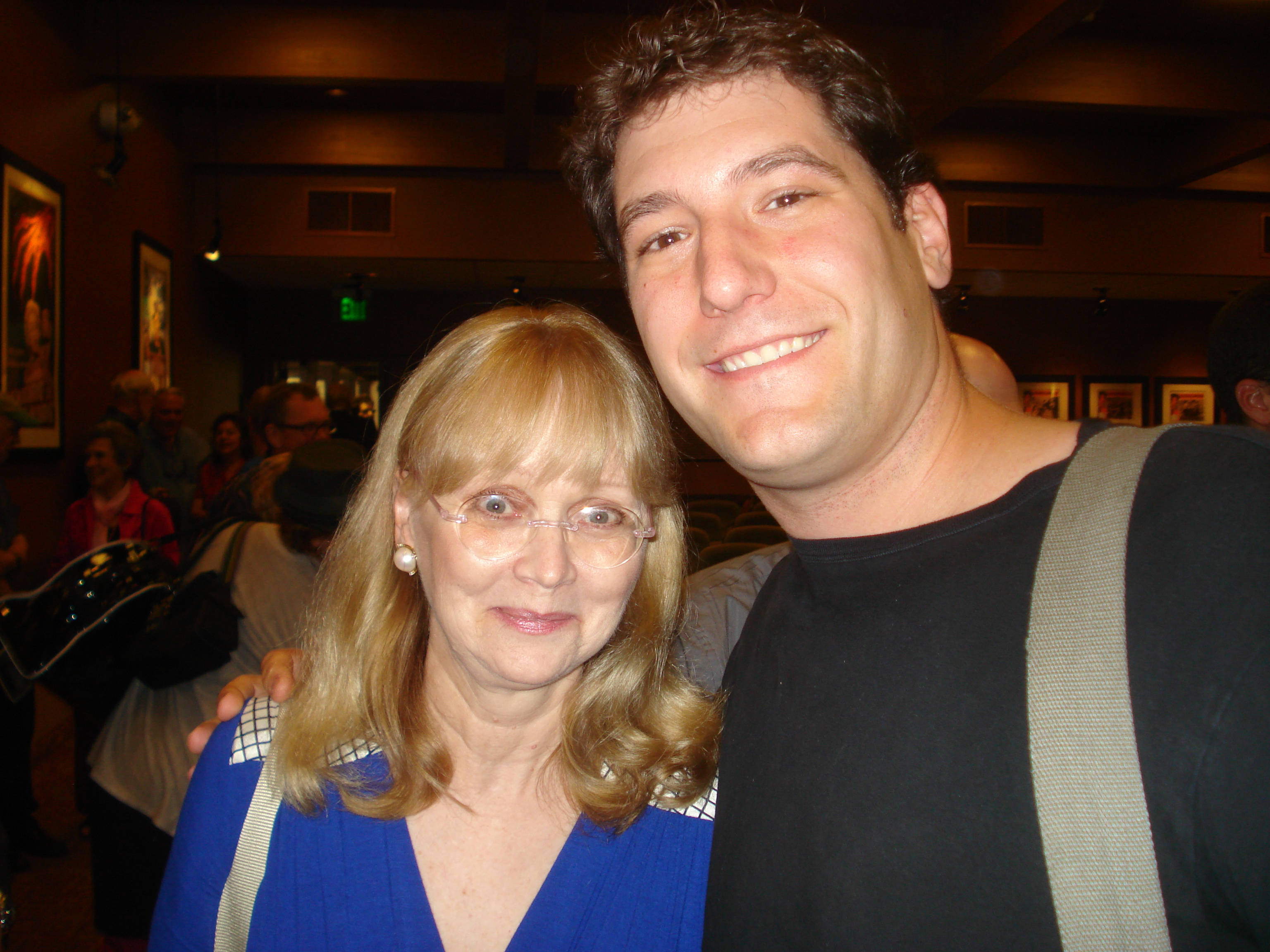This is a photograph capturing the upper parts of two people. On the left is an older woman with shoulder-length honey-blonde hair that slightly covers her right ear. She is looking downwards with her blue eyes, though one description implies a possible discrepancy as it mentions brown eyes. She is adorned with large white pearl earrings, though only the right one is visible due to her hair, and she wears glasses. Her blue v-neck dress features distinctive gold grid-style shoulders, and a strap leading to a bag is seen over her right shoulder. The woman’s facial expression is soft, and she has pronounced cheekbones.

On the right stands a man with wavy dark brown hair that complements his brown eyes, which match exactly. He is smiling warmly at the camera, showcasing the top row of his teeth. His arm is wrapped around the woman's shoulder, adding a sense of connection between them. He is dressed in a black t-shirt and has a nylon strap over his left shoulder, suggesting he's carrying something out of frame.

In the background, the image captures a large indoor room with people milling about, adding a layer of context to the photograph's setting.